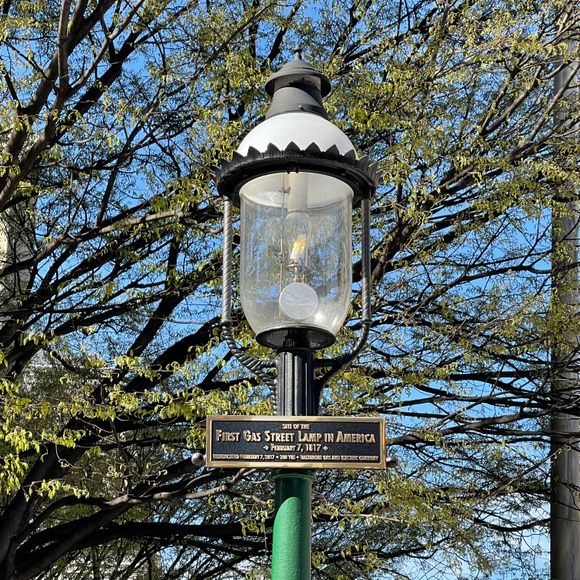The photograph captures a historic gas streetlamp prominently positioned in the center of the frame. The lamp itself features a black-and-white dome-shaped top sitting atop a green lamppost. Below the lamp, a bronze-edged black plaque with gold lettering states, "Site of the First Gas Street Lamp in America, February 7th, 1817." Though difficult to read, more text appears at the bottom of the plaque. The background reveals a backdrop of lush trees adorned with fresh green leaves, suggesting it might be spring. A portion of a building peeks in from the right side, contributing to the outdoor urban scene. Despite being a daylight photograph, the gas lamp appears to be lit. The serene blue sky further enhances the picturesque quality of this historic site.